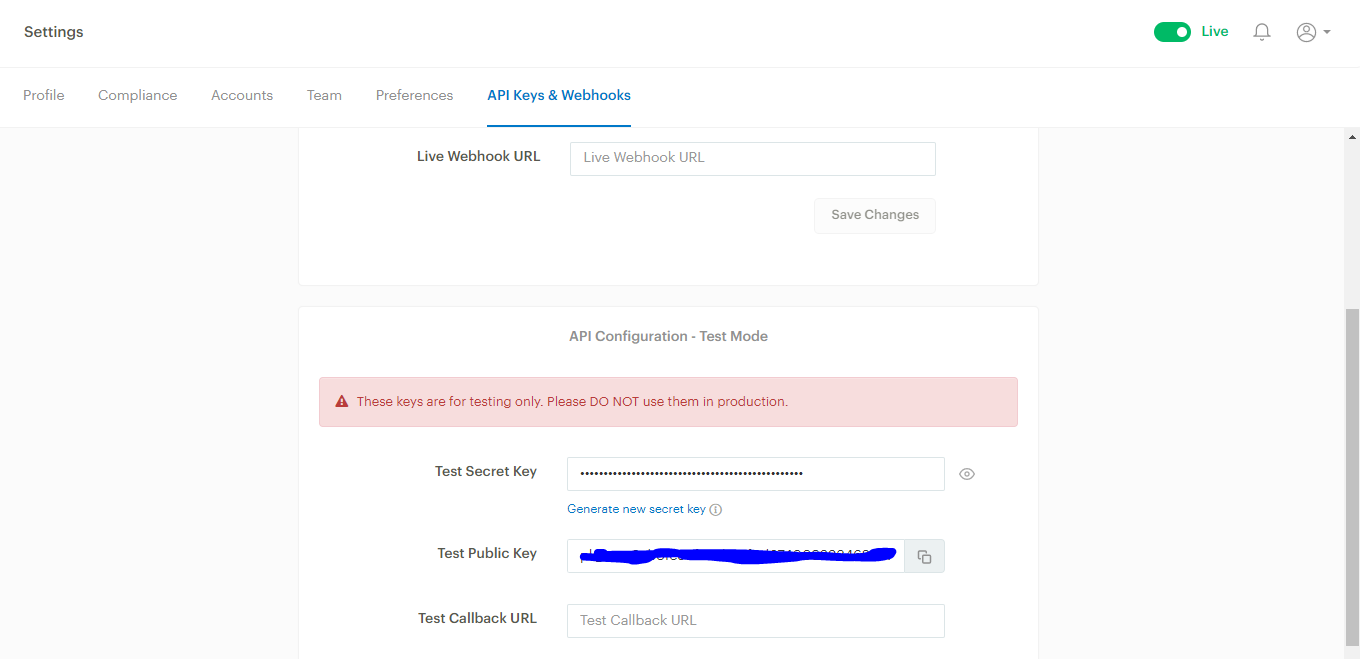In the upper right corner of the interface, a green toggle switch indicates active status. Adjacent to it, a white circle is positioned with the label "LIVE" in green text beside it, accompanied by a bell icon. On the far left side, the word "Settings" is prominently displayed, leading to a list of options below it: "Profile," "Compliance," "Accounts," "Team," and "Preferences." Below these options, highlighted in blue and underlined, are "API Keys" and "Webhooks." Approximately two inches below, in black text, "Live Webhook URL" is noted, followed by a long rectangular input field containing the text "Live Webhook URL."

Below this input field, a button labeled "Save Changes" is enclosed within a box. Further down, the section titled "API Configuration – Test Mode" is displayed. Within a pink rectangle, a red triangle icon accompanies a warning message: "API Keys are for testing only. Please do not use them in production." 

The section continues with fields labeled "Test Secret Key" and "Test Public Key," each followed by a long blue line, which appears to obscure some text. Lastly, the terms "Fast Callback" or "Test Callback URL" are mentioned.